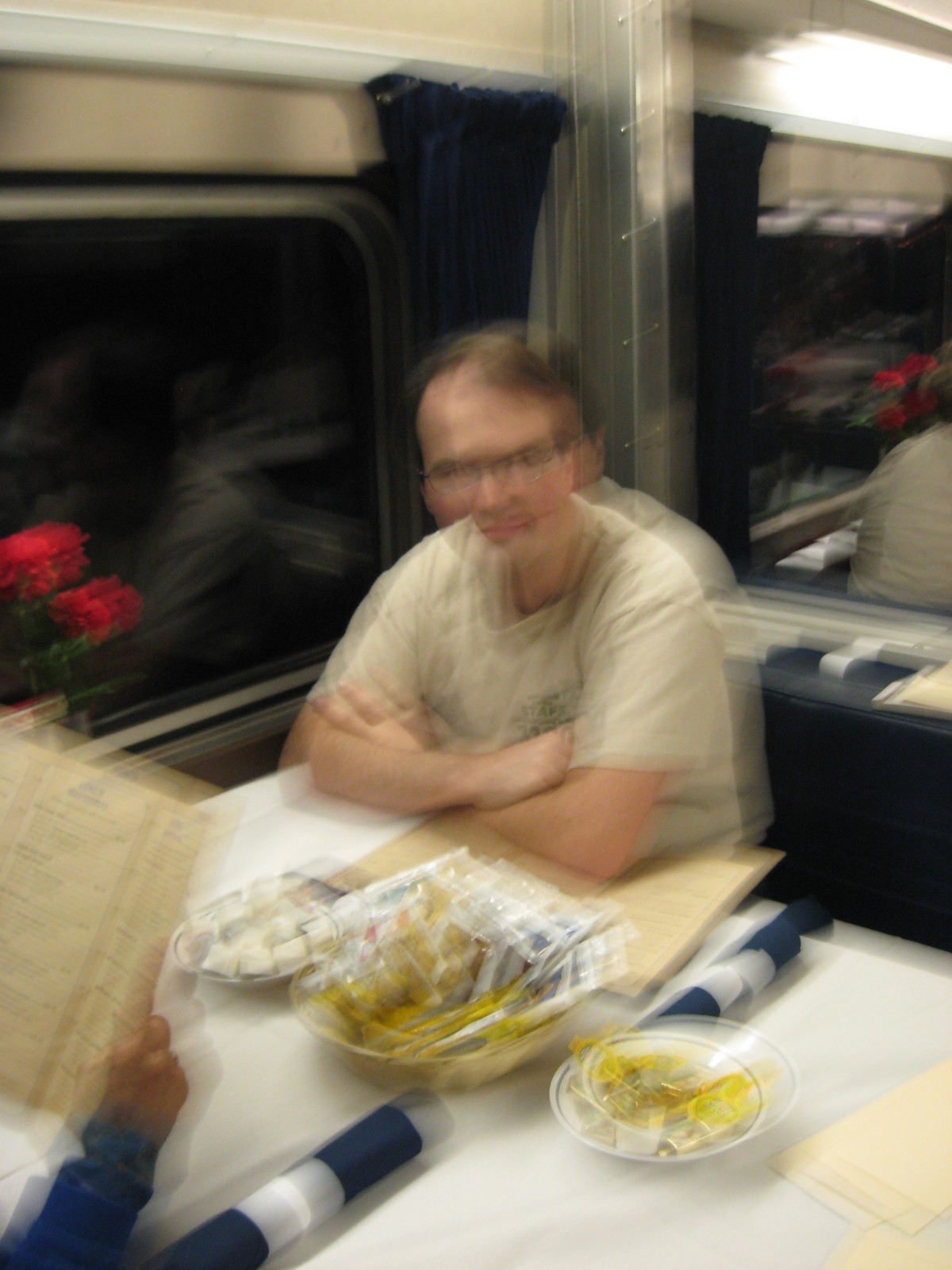In this slightly blurry photograph, a person is seated at a table, seemingly in the midst of a meal. The individual has their arms crossed and gazes directly at the camera, wearing glasses that reflect the ambient light. On the left half of the table, a bunch of vibrant red flowers adds a splash of color to the scene. In the foreground, another person's right hand is seen holding up a menu, partially obscuring their presence. The setting resembles the cozy ambiance of a diner or possibly a dining car on a moving train, which may contribute to the photo's lack of sharpness. While specific details are unclear due to the blur, the image captures a candid moment of dining and the casual atmosphere of the venue.